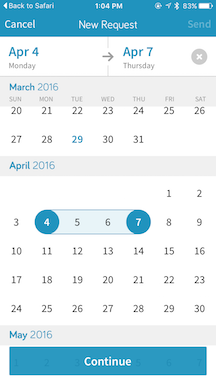Screenshot of a calendar displayed on an Apple mobile device. At the top left corner, an arrow icon indicates the option to return to Safari, the Apple web browser. Below this, the title "New Request" is visible, along with the selected date range "April 4th to April 7th." The partial view of the March 2016 calendar is shown, followed by the April 2016 calendar, where the dates April 4th to April 7th are highlighted. At the bottom, the beginning of the May 2016 calendar is visible, with a blue "Continue" button located beneath it.